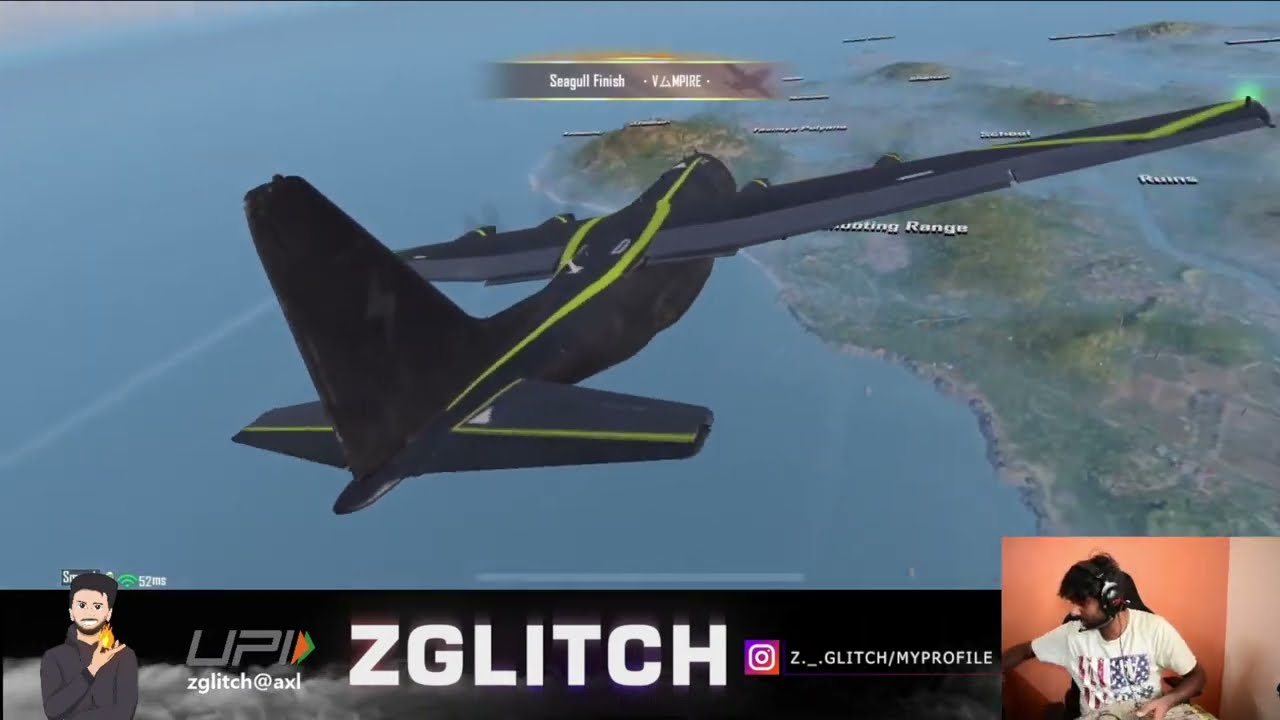This image is an animated screenshot from a flight simulation video game, formatted in a wide, high-definition TV aspect ratio. Dominating the scene is a large, black airplane adorned with yellow and orange-green stripes, flying high above a body of water and approaching a landmass, which features labeled details as if from a map. At the top of the screen, the text "Seagull Finish Vampire" is visible. Below, a black footer contains multiple pieces of information: "UPI", "ZGLITCH at AXL", "ZGLITCH" in large white letters, and the text "z.__GLITCH//myprofile" accompanied by an Instagram logo and an emoji of the player. In the lower right corner, there's a boxed-off, lifelike image of a brown-skinned man in a white t-shirt with a gaming headset and microphone, sitting in a gaming chair and holding a controller, set against a peachy-orange background. The player is looking to his left, deeply engaged in the game.